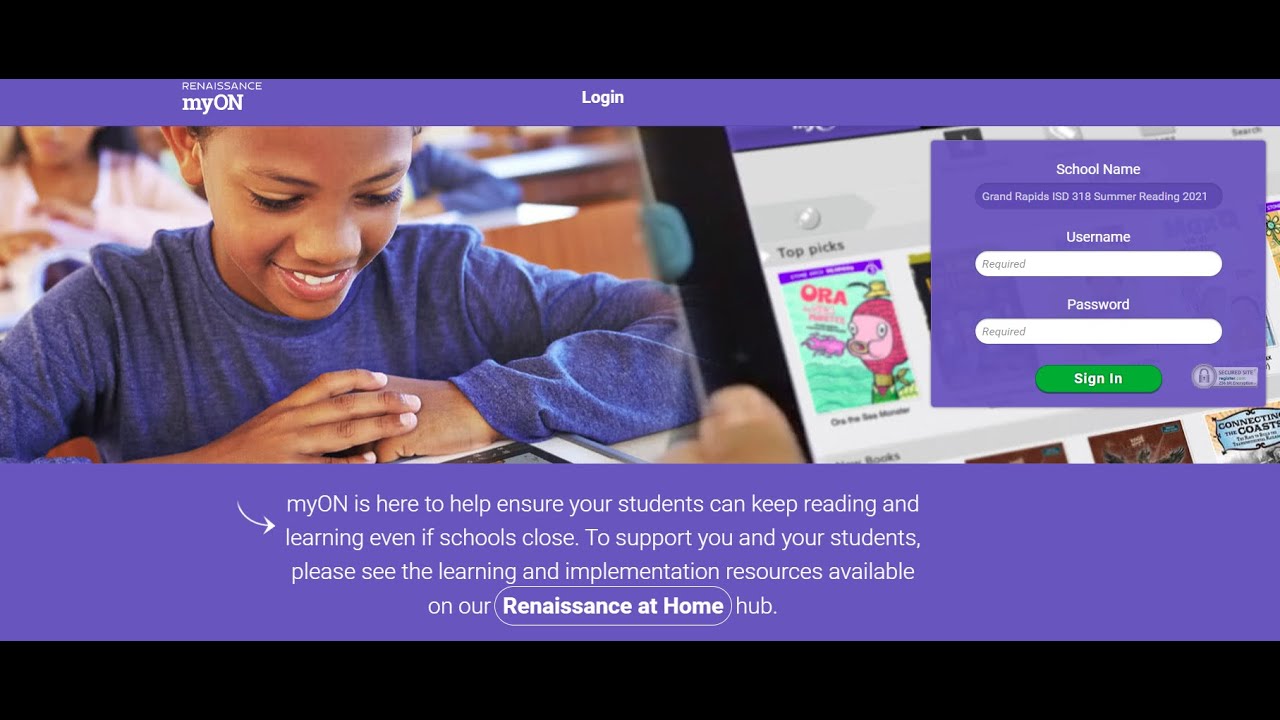The image showcases an educational website designed to facilitate student reading and learning. Central to the image is a young Black gentleman wearing a purple shirt, seated at a desk in what appears to be a classroom setting. He is intently focused on a tablet. To his immediate right, there is a zoomed-in view of the tablet screen displaying a section titled "Top Picks," which likely features a selection of books available for reading on the device.

In the upper left corner of the website, there is a purple-bordered section labeled "Resonant Renaissance MyOn," accompanied by a login button. On the right side of the webpage, there is a section indicating the school name, "Grand Rapids ISD 318 Summer Reading 2021," along with fields to enter a username and password, followed by a green sign-in button.

Below the main image of the young gentleman, a purple bar spans the width of the page, with text emphasizing the utility of MyOn in ensuring that students can continue reading and learning even when schools are closed. It mentions that additional learning and information resources are available on the Renaissance at Home Hub.

Overall, the site appears to be specifically designed to provide children with access to a vast array of reading materials, enabling them to continue their education remotely via a tablet.